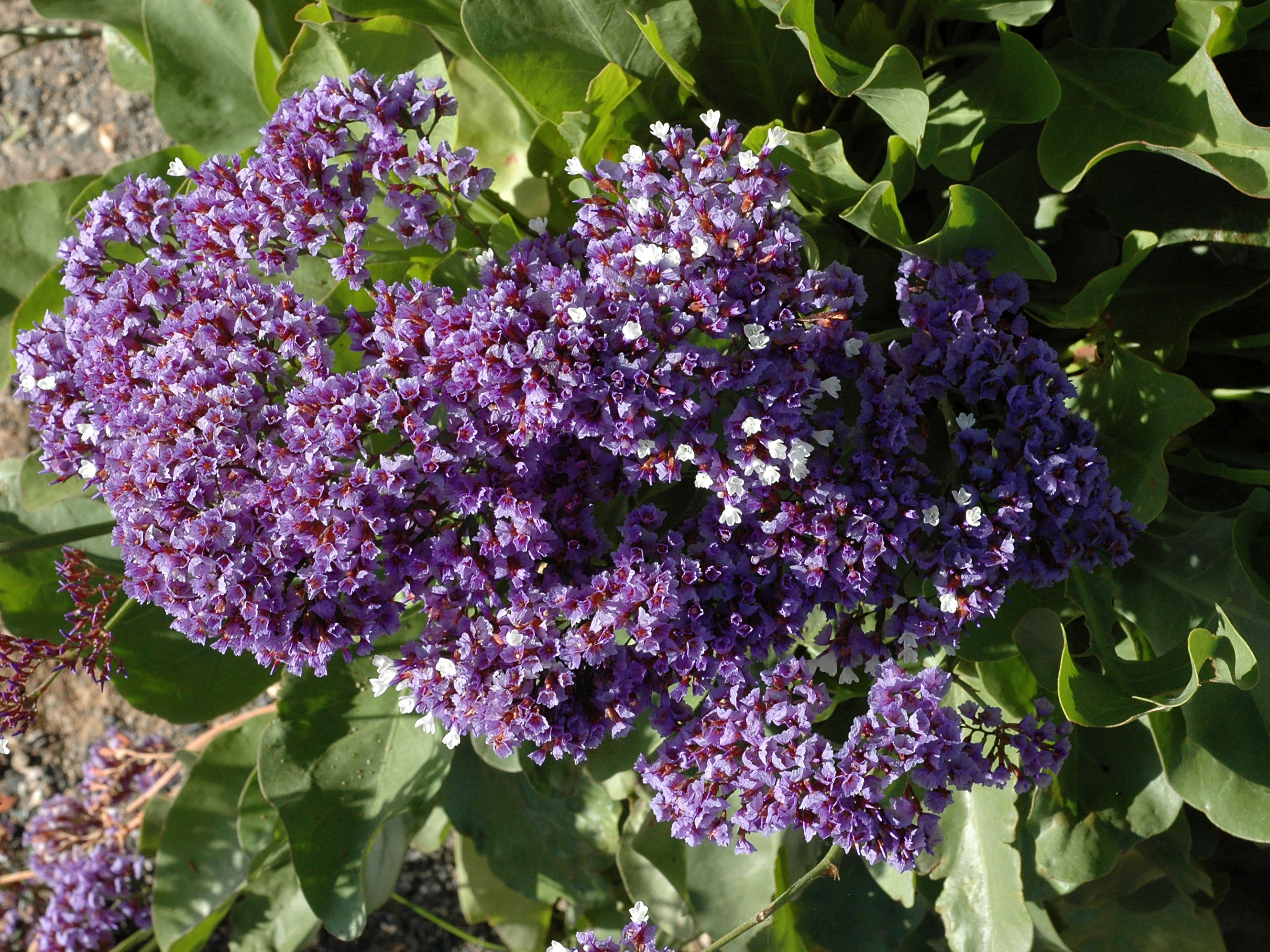The image depicts a lush plant with large, very green leaves that have slightly ruffled edges. At the center of these leaves, a dense cluster of small flowers in varying shades of purple and lilac is prominently featured. Interspersed among the predominantly purple flowers are a few tiny white ones, creating a vibrant mix of colors. Some flowers in the cluster are yet to bloom, with their enclosures showing a striking red color. Intriguingly, the tiny flowers have reddish stems that appear to merge with the petal color, adding an additional layer of complexity to the cluster's appearance. Toward the upper left corner of the image, the green foliage parts slightly, revealing patches of bare ground soil beneath the plant. The overall scene captures the intricate beauty and color variation within this flourishing plant.